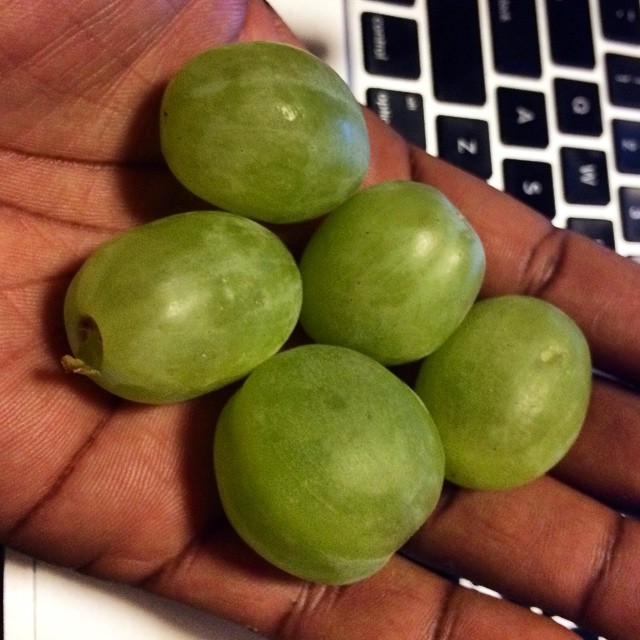In the color photograph, a detailed close-up of a left hand is shown, palm upwards, displaying five green grapes of varying sizes and irregular oval shapes. The grapes, which are plump and fresh with some white patches reflecting the light, are held over a silver MacBook keyboard. The keyboard, oriented perpendicular to the viewer, has black keys with white lettering. The fingers of the hand, though partially cut off at the tips, appear slightly waxy and their back is well visible. A small tear is noticeable on the skin of one of the grapes at the bottom, likely from being plucked off the vine. The hand and grapes, both of which are the primary focus of the shot, rest over the MacBook, with the laptop's silver housing visible in the background.